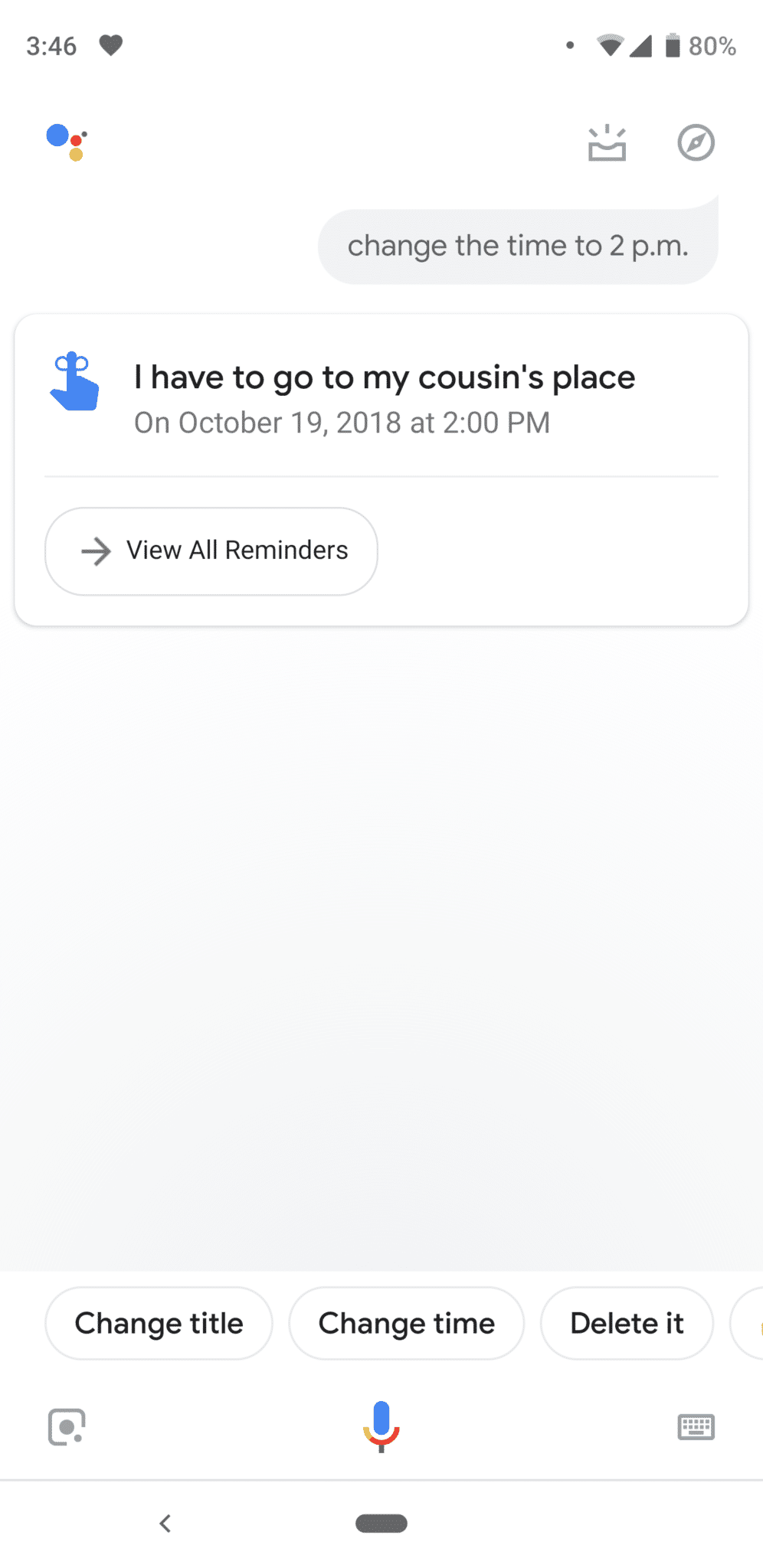The image features a screenshot from a Google app with a white background. In the top left corner, the time "3:46" is displayed in a gradient of light gray to dark gray text. Adjacent to the time, there is a gray filled-in heart icon. The top right corner shows the battery percentage at 80% along with Wi-Fi signal symbols.

Below the status bar, there is a light gray box. To the right of this box, there is an icon resembling Safari's compass symbol. On the far left side of the screen, multiple colored circles in blue, red, yellow, and green are visible.

Directly under the gray box and Safari icon, there's a light gray chat bubble containing black text that instructs, "Change the time to 2 p.m." Below this chat bubble, there is a white box with black text at the top reading, "I have to go to my cousin's place." Underneath this, light gray text indicates, "On October 19, 2018, at 2 p.m." To the left of this text is a blue emoji resembling an upward-pointing finger.

Further down, there is a smaller white rounded rectangular button with "View all reminders" written in black text at the center, accompanied by a right-pointing arrow on its left side. 

At the bottom part of the image, several white bubbles feature different options: the first bubble on the left reads "Change title" in black text, the middle bubble says "Change time," and the bubble on the far right reads "Delete it." Below the "Change time" bubble, a microphone symbol with blue, red, yellow, and green colors is visible.